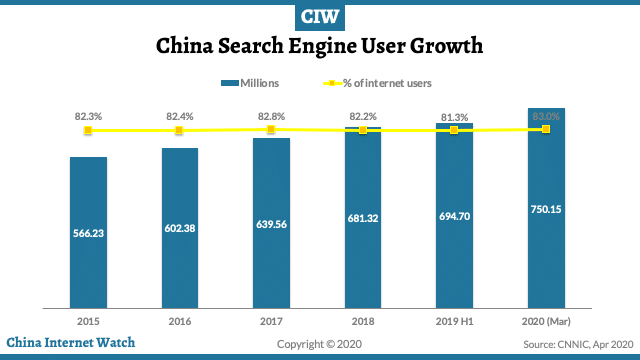This image displays a detailed bar graph depicting the growth of search engine users in China over multiple years. At the top of the image, within a blue rectangular box with white lettering, the acronym "CIW" is prominently displayed. Below this, the title "China Search Engine User Growth" is presented in bold black letters. 

The graph itself differentiates between two key metrics: the number of search engine users in millions (represented by a blue line) and the percentage of internet users (represented by a yellow line).

Here are the data points detailed in the graph:

- **2015:** 566.23 million users, covering 82.3% of internet users.
- **2016:** 602.38 million users, accounting for 82.4% of internet users.
- **2017:** 639.56 million users, representing 82.8% of internet users.
- **2018:** 801.32 million users, translating to 82.2% of internet users.
- **2019 (First Half):** 694.70 million users, comprising 81.3% of internet users.
- **March 2020:** 750.15 million users, making up 83% of internet users.

In the lower left corner, the image credits "China Internet Watch, Copyright 2020," with the source attributed to CNNIC from April 2020.